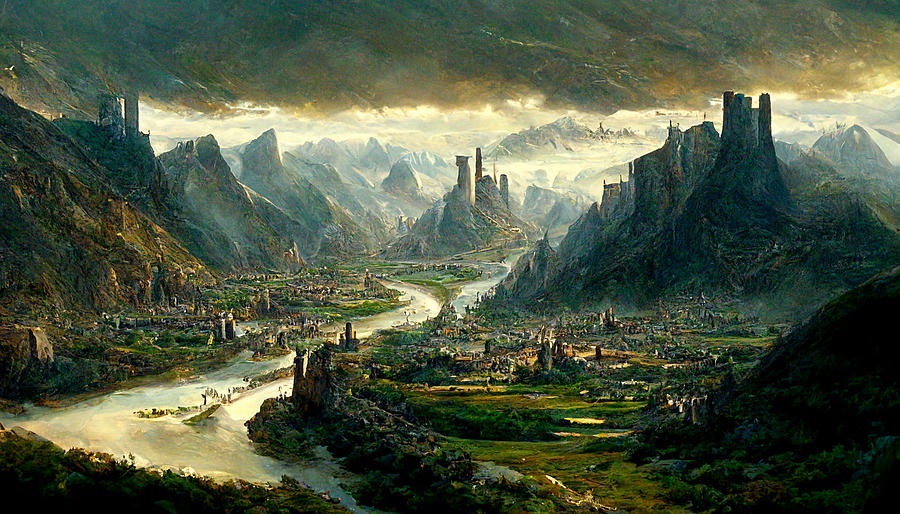This stylistic and detailed drawing portrays a large, fantasy-style city situated in a small valley surrounded by towering mountains with rocky ridges and ominous, misty peaks. The rectangular-shaped city, with its top and bottom sides twice the length of the left and right sides, is bisected by a large, meandering river that starts from the center and flows towards the bottom left corner, eventually transforming into a stunning waterfall. The river is crossed by a small bridge, connecting the two parts of the city adorned with a variety of small buildings and intricate roadways. 

The valley is alive with greenery and fields, lending a peaceful vibe to the area around the river, while the higher elevations are cloaked in dark, stormy clouds casting slight shadows over the landscape. The lush, flat grasslands on either bank of the river feature both farms and residential areas, contrasting with the more industrial city-like buildings on the left riverbank. Further adding to the city's majestic appearance are the tall stone towers and castles situated on the mountain ridges, creating a juxtaposition of medieval and slightly futuristic architectural elements. 

The background is framed by a range of formidable mountains, some of which are white and misty, adding an ominous tone. The sky, while stormy with dark clouds directly overhead, transitions to a serene blue in the distant horizon, suggesting a clash between tranquility and impending turmoil.